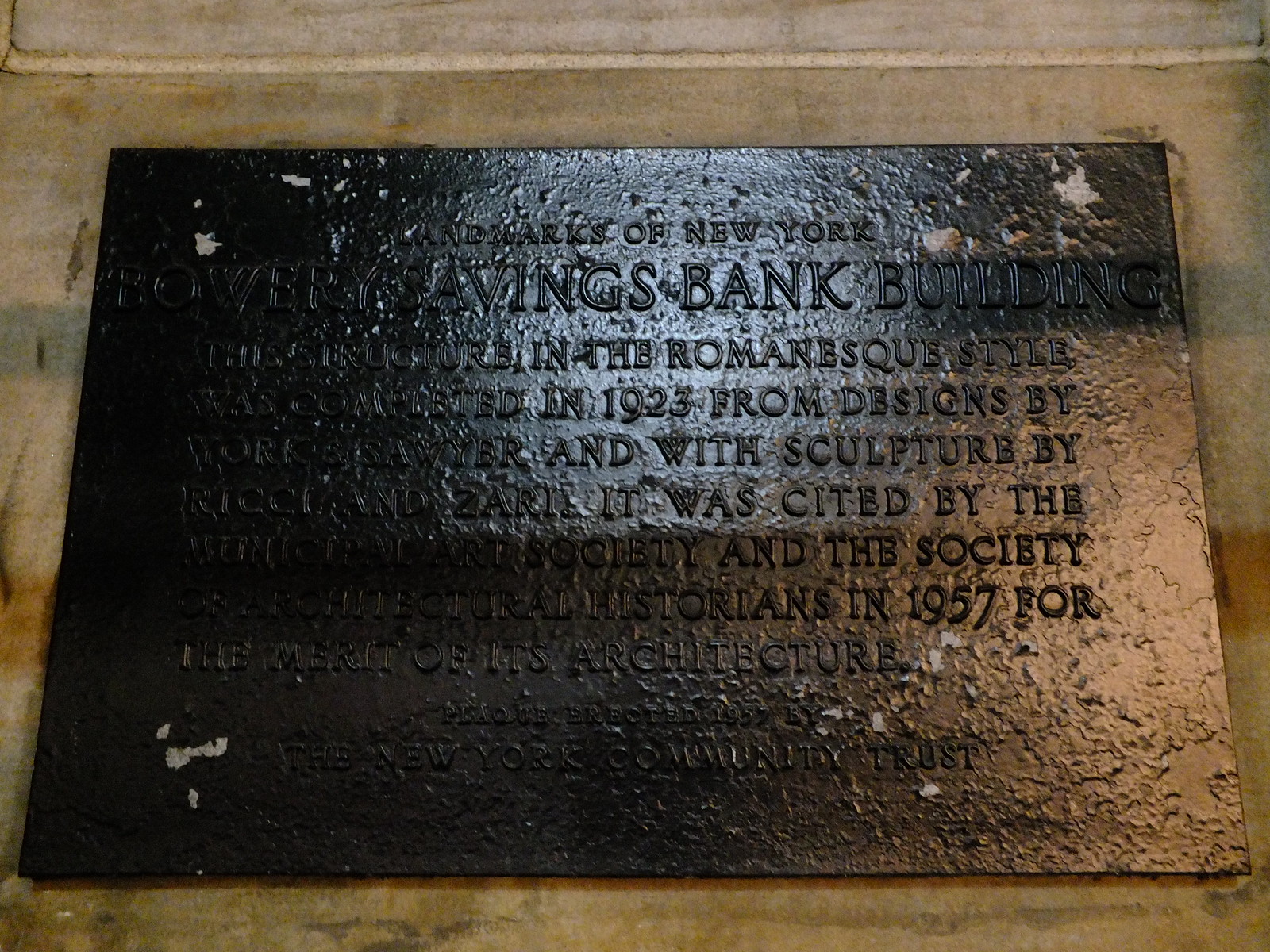This image depicts a black metal plaque with raised engraving, situated on a grayish-beige concrete wall. The plaque, titled "Landmarks of New York," is somewhat difficult to read due to lighting issues which cause certain parts to blur. The most prominent text visible reads, "Bowery Savings Bank Building." The plaque details the building's construction in the Romanesque style in 1923, designed by Works, Sawyer, and featuring sculptures by Rickey and Zari. It was recognized for its architectural merit by a society of historians in 1957. The New York Community Trust is mentioned at the bottom of the plaque. Despite its age and some portions being scratched and chipped, the plaque serves as a dedication to the historical significance of the building in New York.